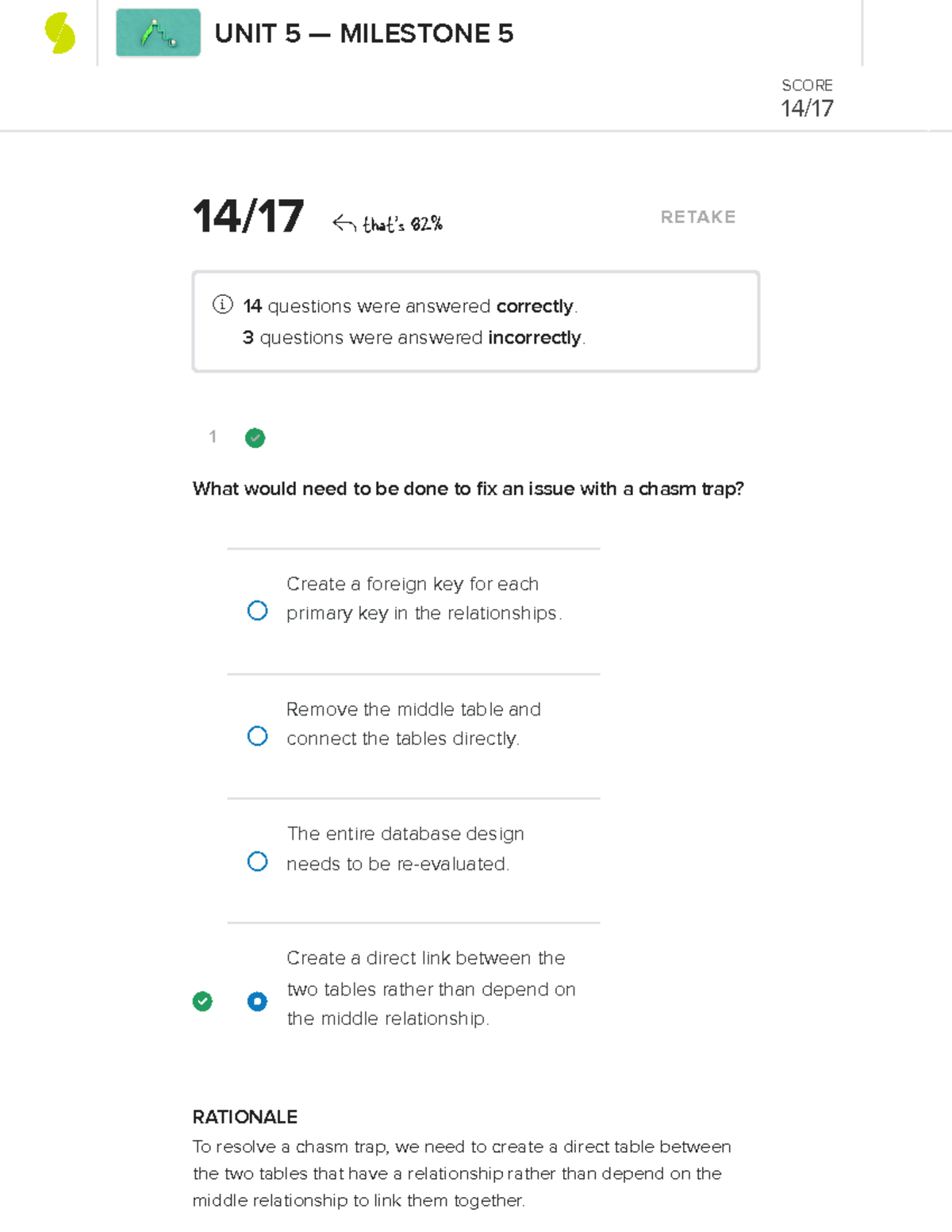In the image, we see a detailed assessment screen for Unit 5. At the top, there are lime green shapes forming what resembles an 'S' structure, created by overlapping a circle and two slightly displaced half-circles. Below these shapes, a teal-colored box features what appears to be a knife or ruler icon. To the right of this icon, the text "UNIT 5 - MILESTONE 5" is prominently displayed in uppercase letters.

On the right side of the screen, there is a score section showing "Score: 14 out of 17," with a vertical line adjacent to the score and a horizontal line underneath. An arrow points leftward from the score, indicating that the result translates to "82%." Below this score section, options for retaking the test and additional information are provided.

A box below this includes an informational icon (a circled "i") followed by the text explaining that "14 questions were answered correctly, 3 questions were answered incorrectly."

The image also displays the first test question labeled "1" with a green circle containing a white check mark beside it. The question is: "What would need to be done to fix an issue with a chasm trap?" The provided answer choices are:
1. Create a foreign key for each primary key in the relationships.
2. Remove the middle table and connect the tables directly.
3. The entire database design needs to be re-evaluated.
4. Create a direct link between the two tables rather than depend on the middle relationship.

The selected answer is the fourth option, indicated by a filled radio button and a green circle with a white check mark. Following the selected option, the rationale is displayed in bold uppercase letters, stating: "To solve a chasm trap, we need to create a direct link between the two tables that have a relationship rather than depend on the middle relationship to link them together."

This caption provides a comprehensive breakdown of the test screen and its elements, detailing both the visual aspects and the content provided.